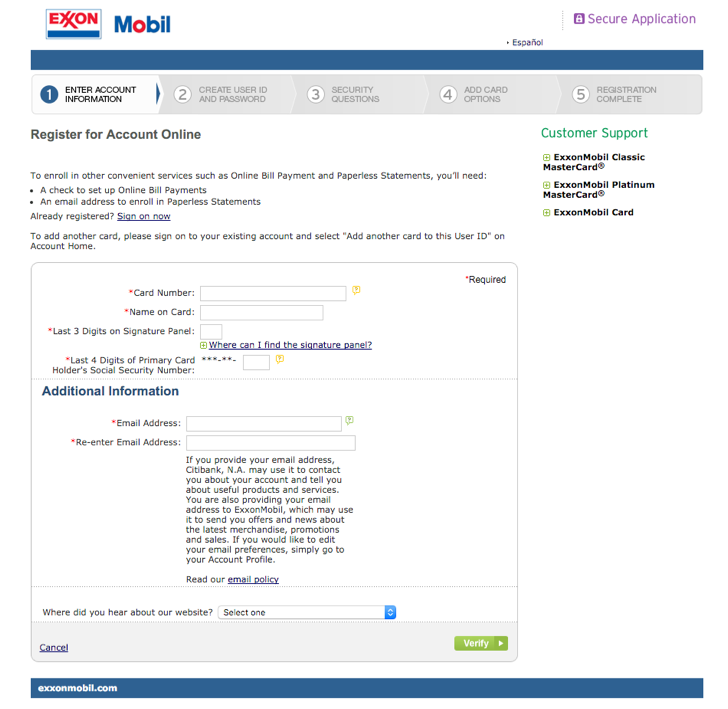**Detailed Caption:**

The image is a screenshot of a website, specifically for Exxon Mobil. The upper left-hand corner prominently features the Exxon Mobil logo. "Exxon" is written in bold red letters, encased within a rectangular box, with a blue line running underneath it. "Mobil" is written beside it, with a blue 'M,' red 'O,' and blue 'B,' 'I,' and 'L.'

The primary color scheme of the website is white, with blue accents. The header section below the logo indicates that the page is intended for users to register for their Exxon Mobil Classic MasterCard account. On the right side of the page, there is a list detailing three types of credit cards that Exxon Mobil offers: the Exxon Mobil Classic MasterCard, the Exxon Mobil Platinum MasterCard, and the Exxon Mobil Card.

Underneath this header, on the left side, there is a section titled "Enter Account Information," which outlines the registration steps: Create a User ID, Security Questions, Add Card Option, and Registration Complete. 

The rest of the page continues with a clean, white background, focusing on a sign-up form. The form includes fields where users should input their card number, the name on the card, the card's last three digits, their email address, and a field to re-enter the email address. There is also a note explaining that the user-provided email address will be used for contact purposes.